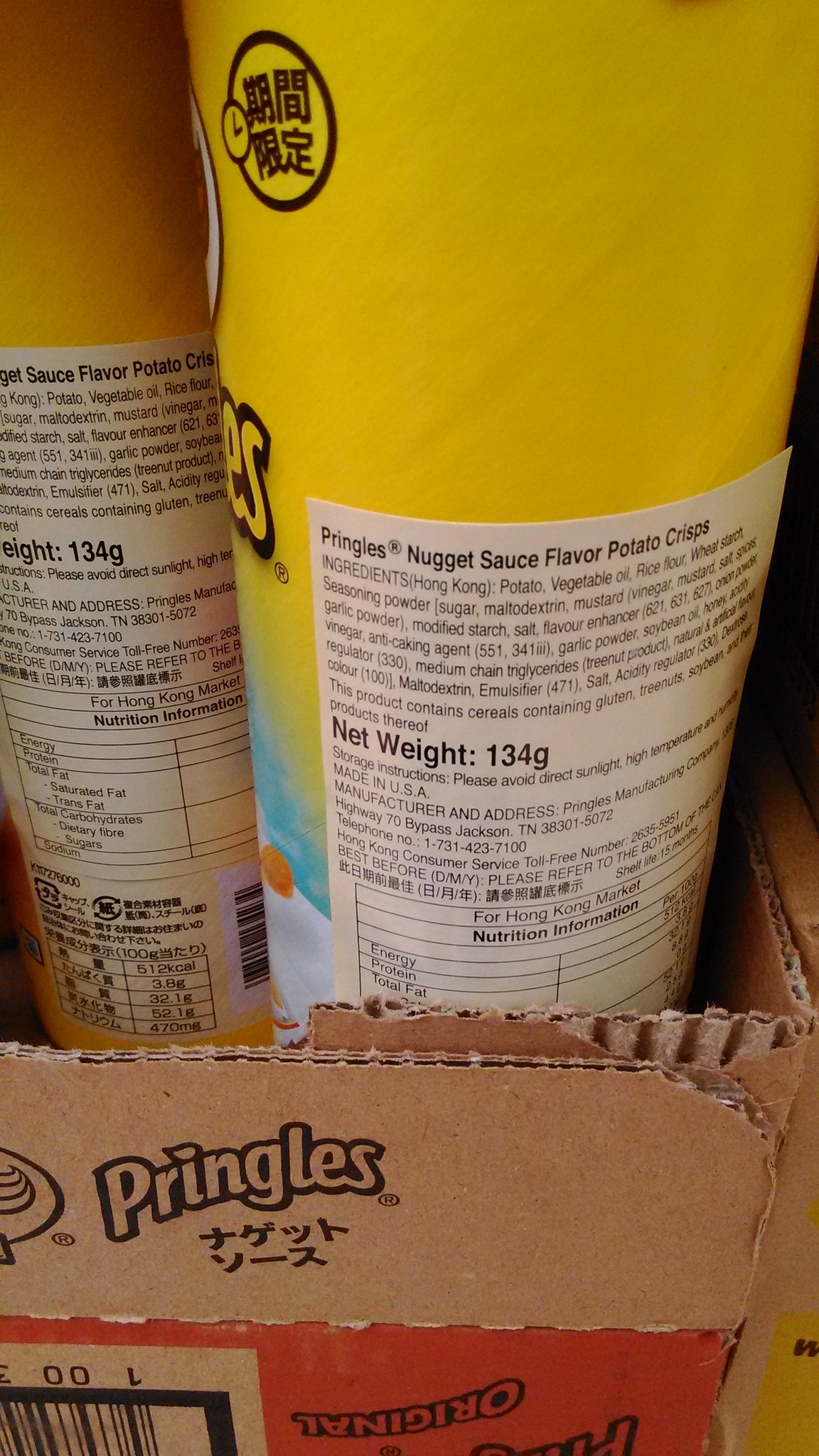The image depicts a brown cardboard box of Pringles situated on a surface, with a zoomed-in view of its contents. The box prominently features the Pringles brand name and some Japanese text below it. A barcode is visible within a brown square, alongside a black line and the number 100 in black. The box also has red details and the word "original" printed upside down in black. Inside the box are two identical Pringles canisters, both displaying the back labels. The canisters are predominantly yellow with some blue and white details at the bottom, partially obscured by the angle. Each canister has a white label that reads "Pringles Nugget Sauce Flavor Potato Crisps" along with the ingredients list and a net weight of 134 grams. Additional text is present on the label, and there is also non-English text printed in a black circle on the canisters.